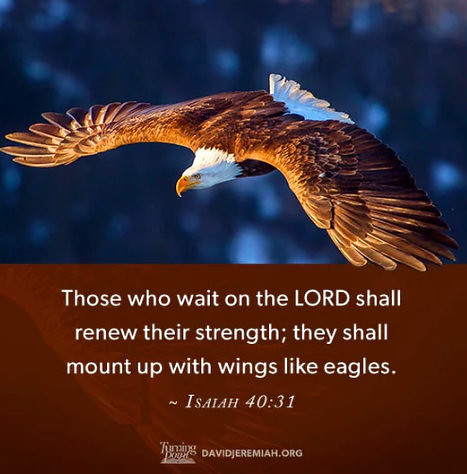The image is a digitally generated poster featuring an inspirational quote. The poster is divided into two sections. The top half shows a majestic bald eagle in flight, its large wings spread wide. The eagle has distinct white head feathers, a striking yellow-golden beak, big brown feathers, and a white tail, flying gracefully against a blurred bluish sky. The eagle's side profile, including its keen eye and talons, is clearly visible.

The bottom section of the image features a brown, melon-colored box with intricate patterns resembling the eagle's wings. Within this box, a quote from Isaiah 40:31 is prominently displayed: "Those who wait on the Lord shall renew their strength; they shall mount up with wings like eagles." Below this quote, at the bottom center, is a logo for "Turning Point" and a reference to "DavidJeremiah.org". The design and layout suggest it is intended for social media sharing, likely on platforms such as Twitter or Instagram.